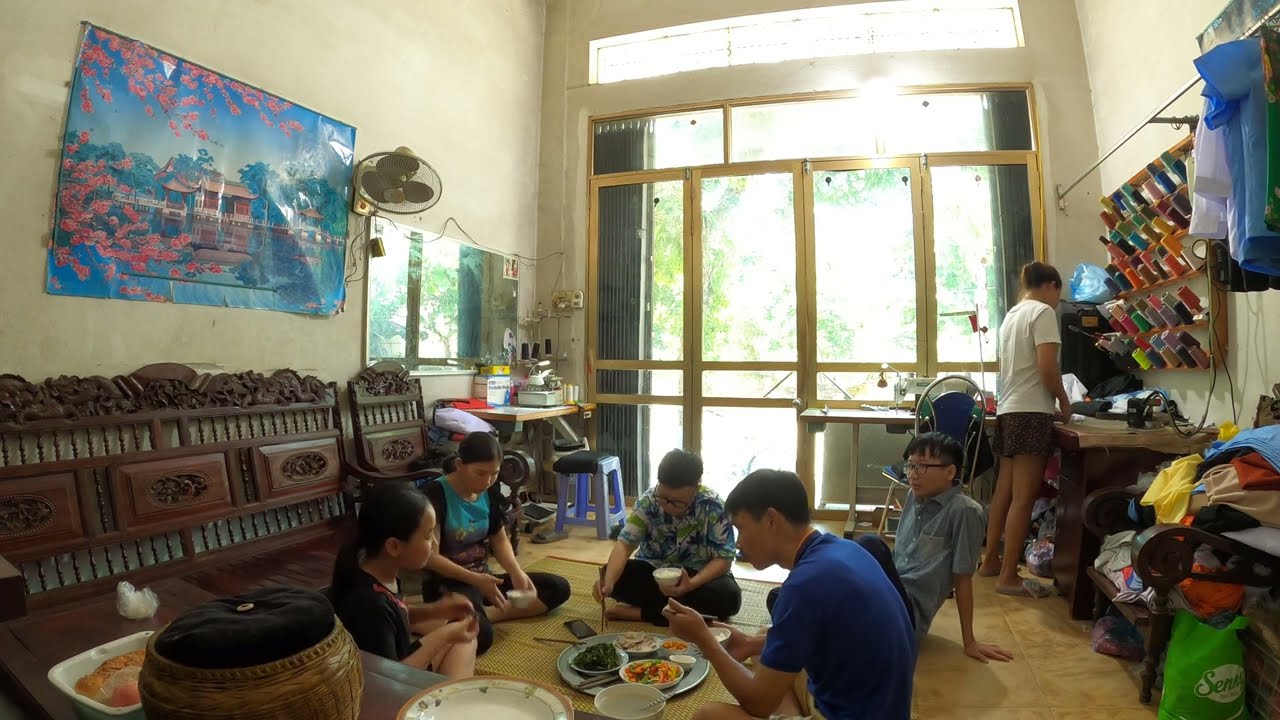In this detailed photograph, we see a group of five Asian people seated on a bamboo mat around a large circular silver tray laden with various dishes, which include black-colored food, bread, orange-colored fruits, and possibly meat. The gathering is taking place inside what seems to be a home or a dorm-like setting with a slightly disheveled appearance. The walls are off-white, and there is a prominent glass door with gold frames leading to the outside, allowing sunlight to stream in and illuminate the room.

On the left side of the image, behind two women sitting cross-legged, is an ornate wooden bench and a chair. Above them hangs a blue and pink poster depicting a serene lake surrounded by cherry blossom trees with a temple in the background. Further left, a mirror is visible near the window, and a mounted fan can be seen on the wall to the right of the poster.

In the center, a man faces the camera, engaged in the shared meal. To his right, another two men participate in the gathering. Meanwhile, a woman stands to the right of the group, beside a desk, appearing to adjust something on it—perhaps involving food or a computer. Above the desk, spools of colorful thread or yarn are organized on racks. In the bottom right corner, a wooden chair is cluttered with various colored clothes or fabrics, and a green cloth bag rests on the floor in front of it. A bright blue stool with a black cushion also peeks into the scene from behind. The room speaks of a casual, lived-in environment where friends or family are enjoying a communal meal amidst the everyday hustle.